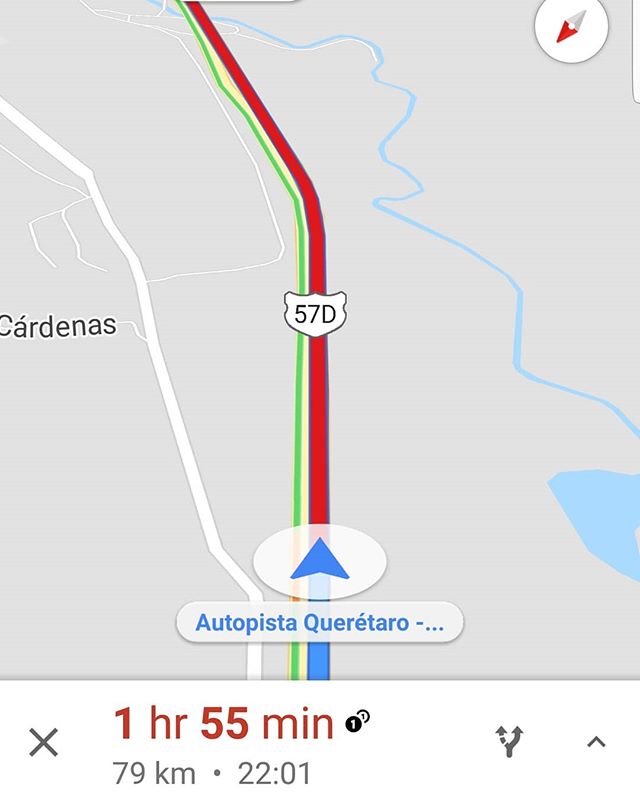The image displays a detailed map on a digital screen, either from a computer or a phone, resembling a Google Maps interface. Dominating the map is a road labeled Autopista Queretaro, which starts as a thick blue line at the bottom and transitions to red as it moves upward and slightly to the left. Prominently in the center, there's a highway marker for 57D. To the left, near the junction where the color changes, the word Cardenas is visible in black lettering.

On the surrounding map, winding through in the upper portion, there is a blue river that flows in a zigzag pattern from the right. Adjacent to this is a green line signifying another route, which angles off to the left about two-thirds up the map. Below this, at the bottom left, a black "X" marks a significant point, accompanied by a red text indicating a travel time of 1 hour 55 minutes. Beneath that, black text signifies the distance as 79 kilometers, followed by the number 2201.

A series of icons and labels further detail the map: a prominent white oval with a blue arrow points up the road where the blue color changes to red, and a white oblong label with blue text spells out AUTOPISTA QUERETARO. The color scheme of the map also features light bluish and pinkish hues, contributing to a modern, digital appearance.